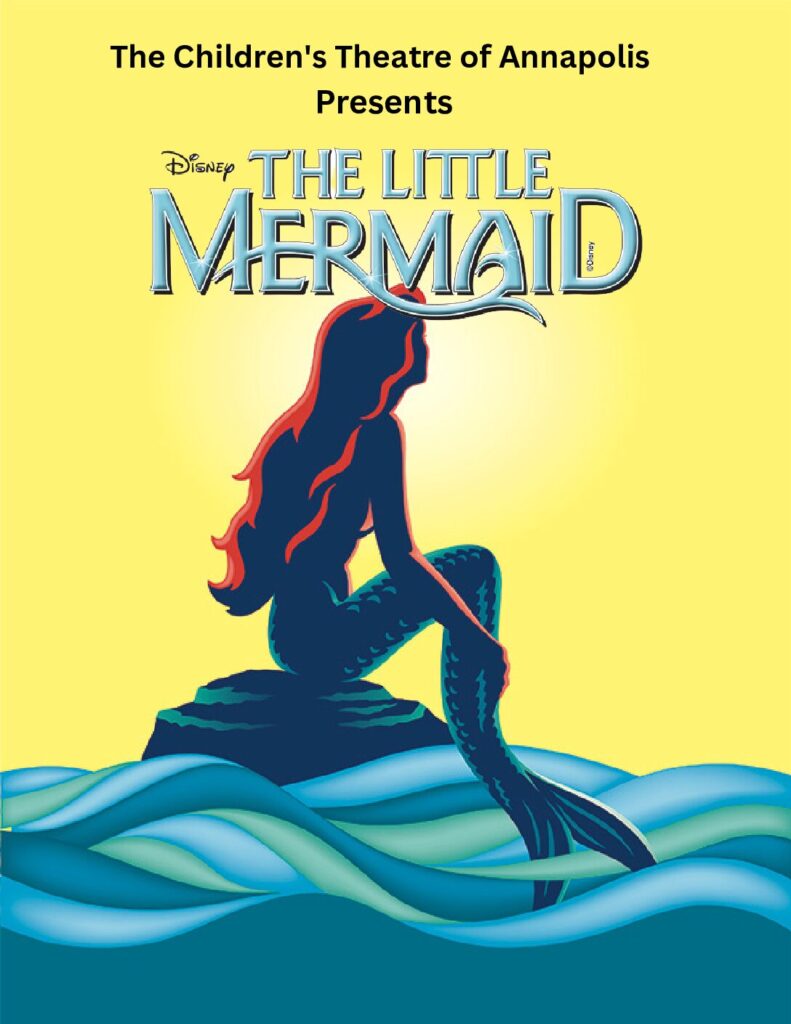The poster for "The Little Mermaid," presented by the Children's Theatre of Annapolis, features a striking silhouette of Ariel. At the top of the poster, in black letters, it reads "The Children's Theatre of Annapolis presents Disney," with "Disney" penned in its classic script. The title "The Little Mermaid" is rendered prominently in large blue letters. Ariel is depicted in a black silhouette with a distinctive red outline capturing her flowing hair. She sits on a prominent rock that juts above the ocean surface, her tail partially submerged. Ariel's knees are bent as she wraps her arms around her tail, gazing upward towards the sky. In the background, a faint silhouette of the sun peeks through a golden-yellow sky. The water beneath the rock is alive with blue and green hues, interspersed with lighter streaks, creating the effect of waves. The overall design exudes a painted or pastel animation style, making it visually engaging and vibrant.